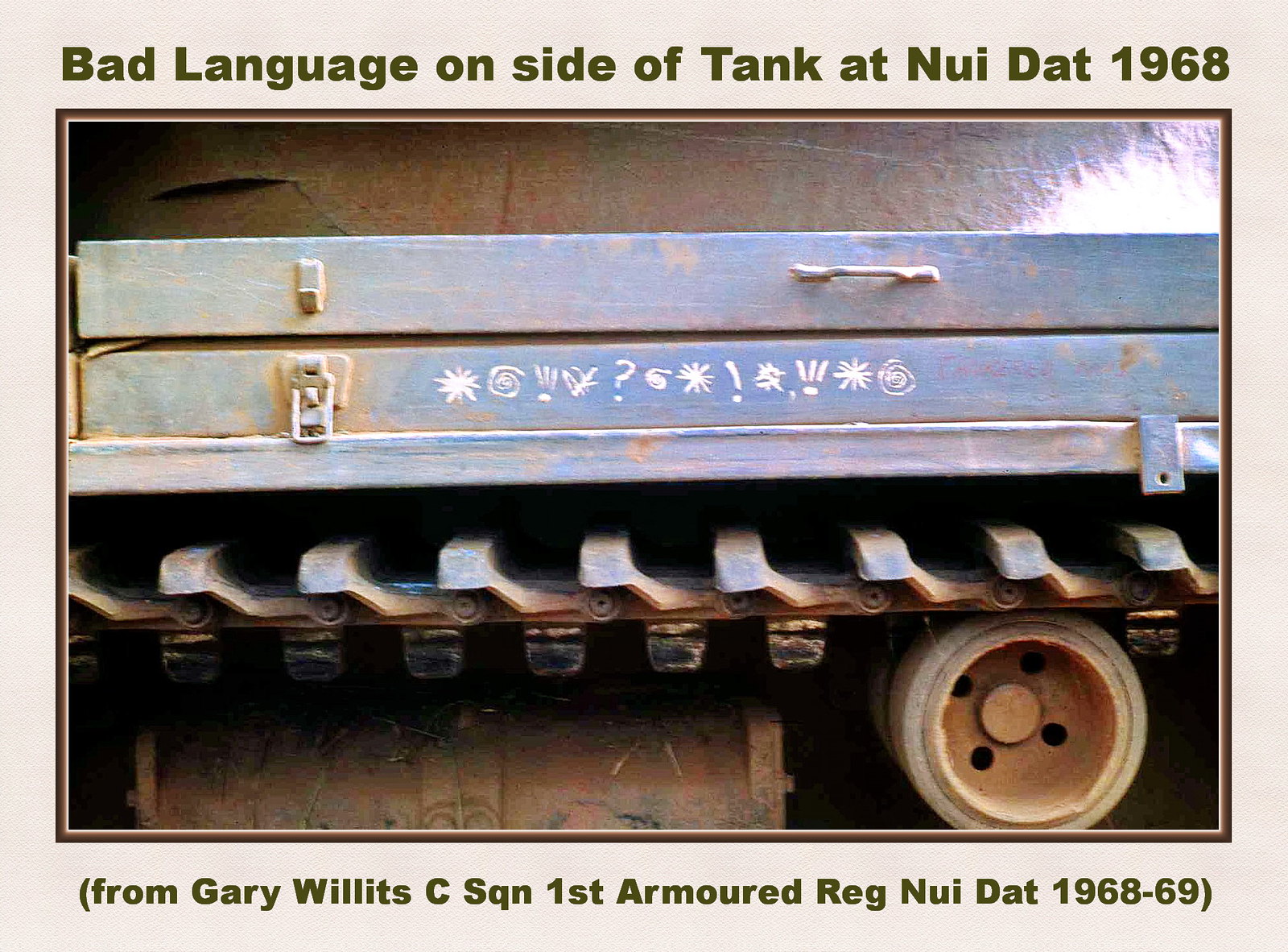The image, taken in 1968-69 and framed with pinkish paper and a brown border, is titled "Bad Language on Side of Tank at NUIDAT, 1968," as indicated by green text at the top. Below the image, a note in parentheses reads, "From Gary Willits, C.S.Q.N., First Armored Regiment, NUIDAT, 1968-69." The photograph depicts the side of a rough-looking tank, which, curiously, has wooden panels giving it an appearance somewhat akin to a wagon or trolley. One panel, which appears to have a handle and a latch akin to that of a toolbox, is adorned with white graffiti-like symbols, including a star, spiral, exclamation point, and question mark. The lower section of the image features what looks like a metal tread with teeth and a wheel on the lower right-hand side. The tank, painted baby blue, defies the typical image one might have of armored military vehicles, adding to its unique and historical significance.